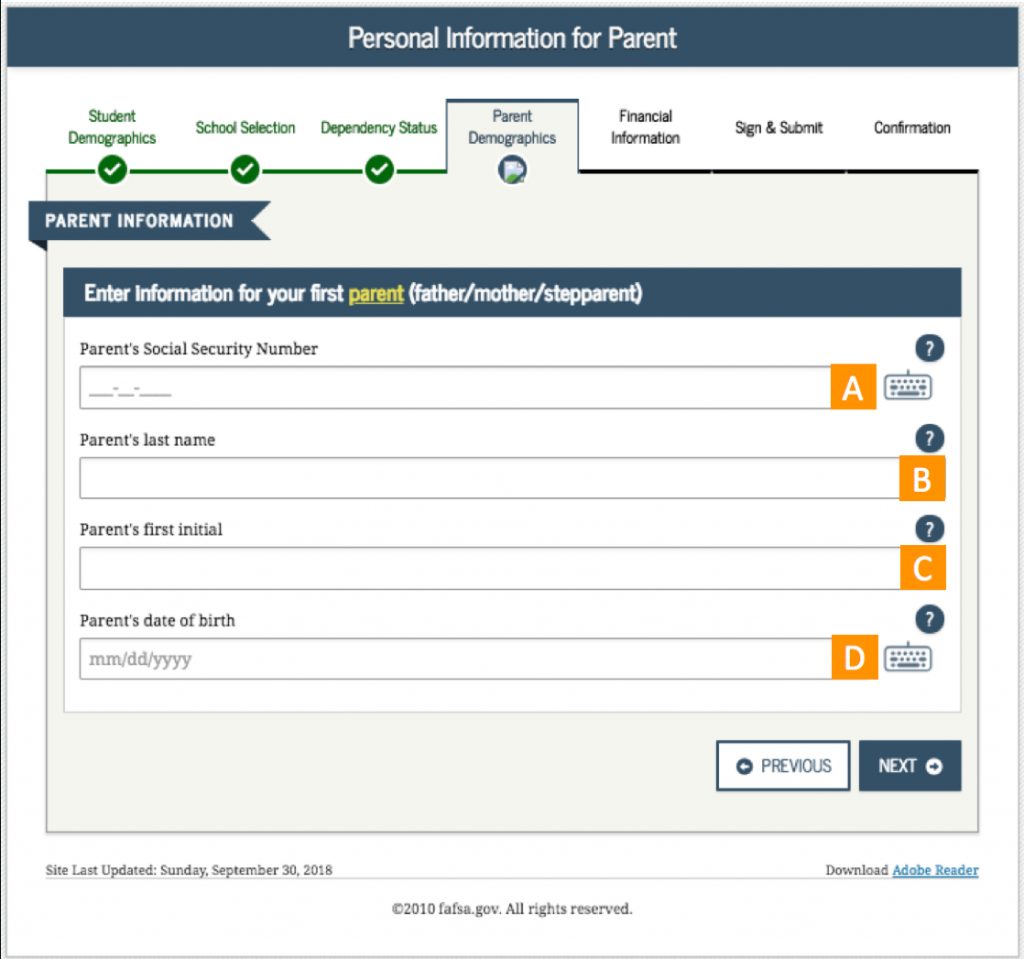This image is a screenshot of a website interface displaying a section dedicated to entering personal information for a parent. The page features a dark blue banner at the top, with the header "Personal Information for Parent" prominently displayed in white text, with each important word capitalized. 

Directly beneath the banner, the background switches to white, contrasting with green text that reads "Student Demographics." Below this text, there is a circular icon with a white checkmark inside. Sequential sections include titles such as "School Satisfaction," "Dependency Status," and "Parent Demographics," with the latter written in blue text.

Continuing down the page, several more section titles are presented in black text, including "Financial Information," "Sign and Submit," and "Confirmation." 

Further down, another blue banner appears, again using white text to display "Parent Information." Below this, a section with a blue background and a blue banner advises the user to "Enter Information for Your First Parent" with the word "Parent" highlighted in yellow-green text. In parentheses, the text clarifies acceptable entries: "Father / Mother / Step Parent."

Underneath this directive, there is a white input form listing several fields for data entry: "Parent Social Security Number," "Parent's Last Name," "Parent's First Initial," and "Parent's Date of Birth." At the bottom, navigation buttons labeled "Previous" and "Next" allow users to move through the form.